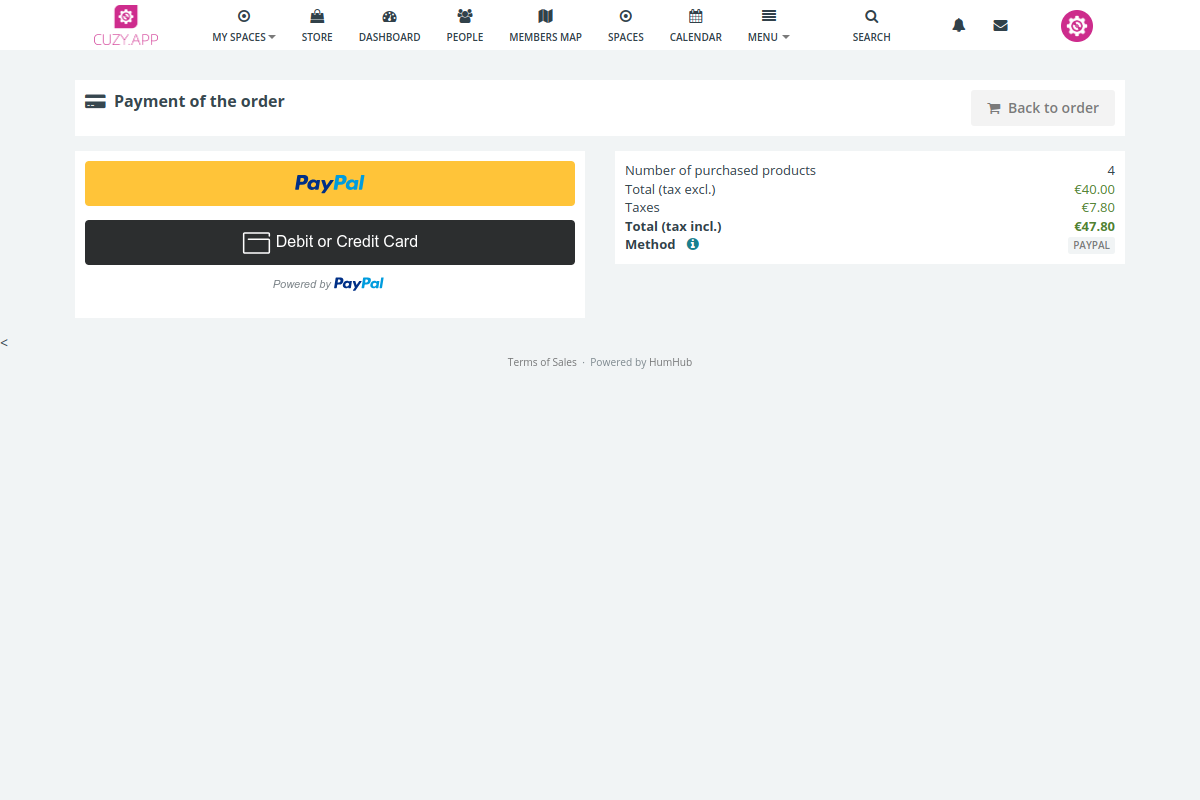The image appears to be a screenshot of a web interface, possibly for an e-commerce or social platform. The top bar includes various icons: a red square with a gear icon representing settings, and icons for "My Spaces," "The Store," "The Dashboard," "People," and "Members Map." Also present are "Spaces," "Calendar," and a "Hamburger Menu," which presumably opens additional options. The platform is named 'Symmetrica,' as indicated by the branding.

To the right, there are search, notification (bell), and message (envelope) icons, all designed in a cohesive visual style. The middle section of the page provides details about a recent transaction: 

- A white rectangle housing the primary transaction details.
- A gray rectangle with a "Back to Order" button. 
- A yellow rectangle indicating the PayPal payment option.
- A black rectangle displaying the option to pay via "Debit or Credit Card," also powered by PayPal.
- Transaction details beneath include the number of purchased products, which is four, 
  - Total tax-exclusive amount: €40,
  - Taxes: €7.80,
  - Total tax-included amount: €47.80,
  - Payment method: PayPal.

The page footer contains the text "Powered by HumHub," twice, and appears on a gray background.